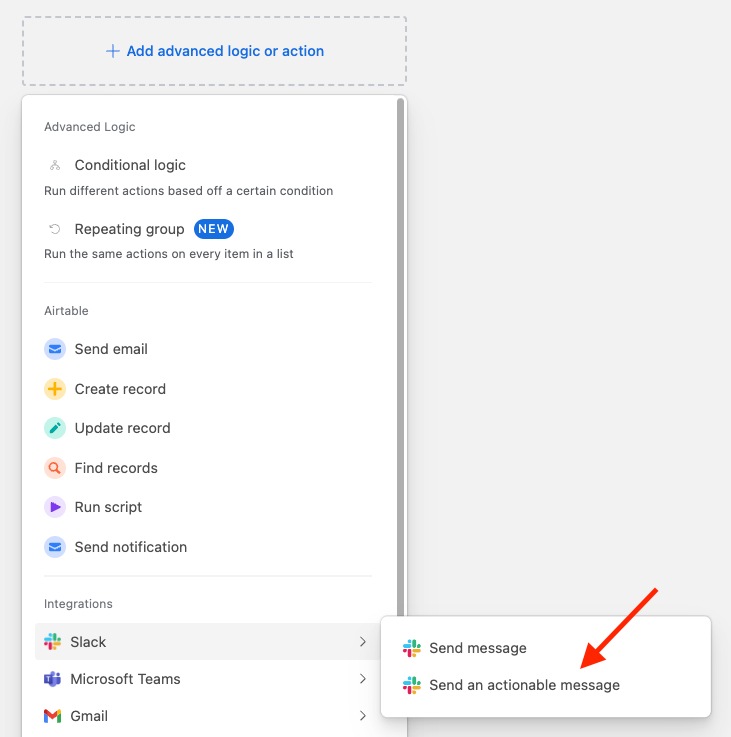In the image, we see a screenshot from a software or program, depicting a user interface for setting up advanced logic or actions. At the top, there's a prominent plus button labeled "Add Advanced Logic or Action." Below this, a dotted rectangular placeholder suggests an area where new logic or actions can be added. 

Underneath this section, there are several categorized options. The first category, "Advanced Logic," features options such as "Conditional Logic" and "Repeating Group," indicating functionality for sophisticated logic configurations.

The next section is dedicated to "Airtable," with possible actions including "Send Email," "Create Record," "Update Record," "Find Records," "Run Script," and "Send Notification," highlighting its extensive integration capabilities.

Finally, under the "Integrations" category, we see options for integrating with various applications. The listed integrations are "Slack," "Microsoft Teams," and "Gmail." At this moment, "Slack" is selected, as indicated by a highlighted and focused state. A red arrow points down to the option "Send an actionable message," suggesting the user is in the process of configuring this specific Slack action.